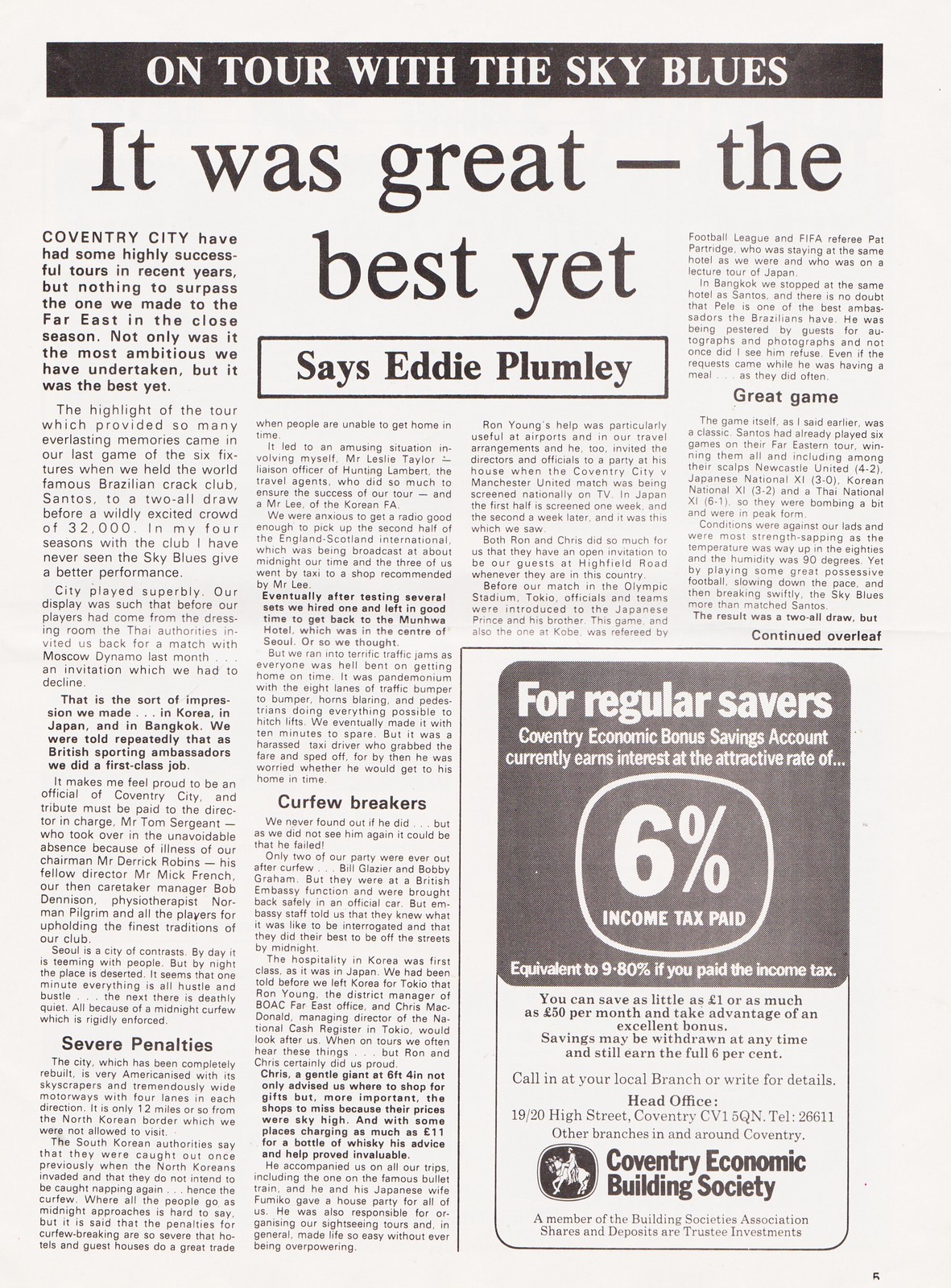The image depicts a page from an old newspaper. At the top of the page, a black banner with white lettering reads "On Tour with the Sky Blues." Below this, in large black letters, the headline states "It Was Great – The Best Yet," with "Best Yet" centered under the word "Great." Beneath the headline, within a white box outlined in black, the name "Eddie Plumlee" is prominently displayed. The article spans four columns of very small text, featuring bold headings such as "Severe Penalties," "Curfew Breakers," and "Great Game." The bottom right-hand section contains an advertisement for Coventry Economic Building Society's Bonus Savings Account, which highlights a 6% interest rate with income tax paid. The page also includes a reference to Coventry City's successful tour to the Far East, adding context to the historical and sports-related content.